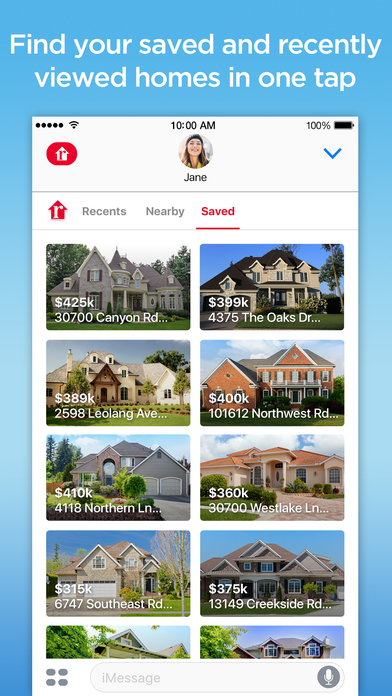The image is a screenshot from a real estate site displayed on a cell phone screen with a portrait orientation. The screen features a light blue background with white text at the top that reads, "Find your saved and recently viewed homes in one tap." Below this, still on the blue background, there is an inset image that simulates another cell phone screen.

The simulated cell phone screen is predominantly white and shows various interface elements. In the top left corner, there are five dots, accompanied by a wireless signal icon. The center of this simulated screen displays the time as 10 a.m., and the top right corner shows a battery icon at 100% charge.

On the left side of this simulated screen, there is a filled red oval with a lighthouse and a red "R" in it. Adjacent to this, in the middle of the second line, there is a profile picture of a woman with light skin and long dark hair, labeled as "Jane." To the right of her image is a downward-facing blue caret.

Moving down the screen, the next line begins with a red house icon featuring a white "R." Following this, it says "Recent" in gray, "Nearby," and "Saved" in red and underlined, indicating that the current view displays saved information.

The main content of the screen is organized into four and a half rows and two columns, clearly showing eight full squares and the top halves of two additional squares in the fifth row. Each square contains a color photo of a beautiful, spacious house along with its price, which ranges from $315,000 to $425,000, and the address of the property.

At the bottom of the screen, there are four gray dots, an iMessage text field, and a microphone icon on the right, likely indicating navigation or additional functionality.